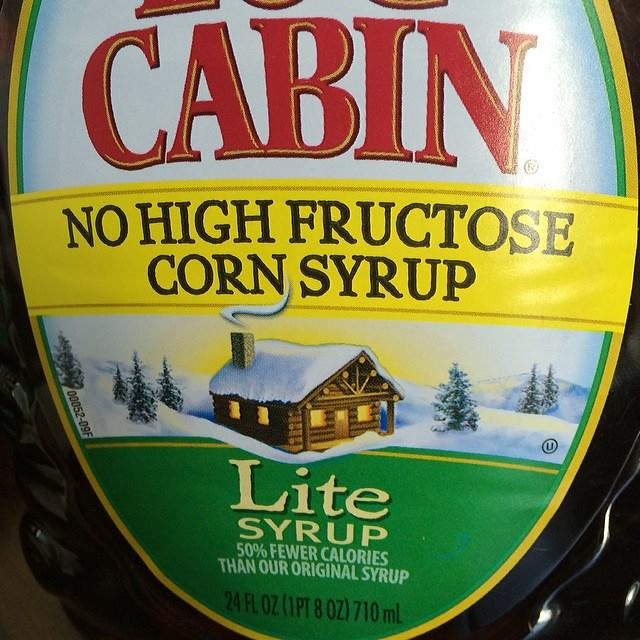This detailed photograph showcases a bottle of Log Cabin Maple Syrup, packaged in a clear plastic bottle. At the top of the label, the brand name "Log Cabin" is prominently displayed in bold red font. Directly beneath, in black text, the label highlights the absence of high fructose corn syrup in the product.

Taking center stage on the label is a warm illustration of a classic log cabin. The cabin, crafted from lighter-toned wood, features a chimney and a roof blanketed in snow. Warm amber light glows from within the cabin, creating a cozy contrast against the snowy backdrop, which includes snow-covered trees.

Further down, the label informs consumers that this is a "Light Syrup" with 50% fewer calories than the original version. This information is presented in green with white font. Near the bottom, the quantity is clearly specified in black text: 24 fluid ounces (710 ml). Additional details, such as black numbers and a black 'U' symbol, are subtly visible against the snowy background on either side of the label. The photo boasts crisp clarity, allowing viewers to see fine details and subtle light reflections at the bottom of the bottle.